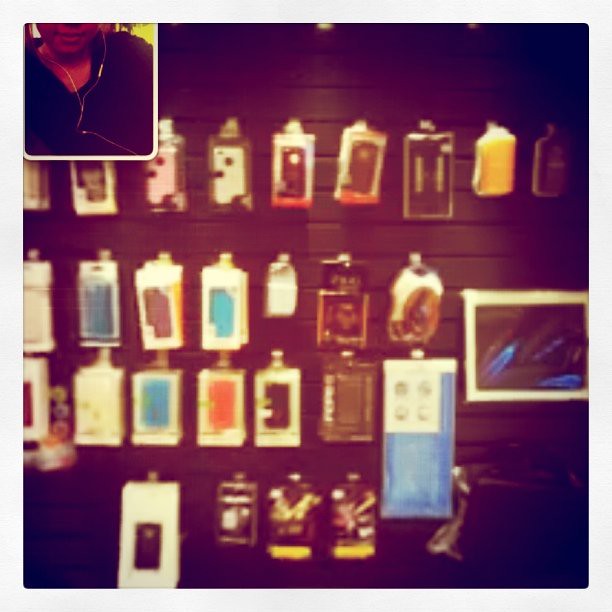The image is a very blurry photograph of a cell phone store display. The overall photo is framed by light gray borders, with an additional white-bordered thumbnail in the top left corner showing a cropped image of a person, visible only from the mouth to their chest. This individual, who appears to be a woman, is wearing headphones and a black t-shirt, with a wire hanging down their chest. The main display wall is a slatted board, allowing for metal hooks to be inserted to hold various products. Hanging on these hooks are an array of items, including phone cases, screen protectors, and cables, though the image quality makes it challenging to distinguish them clearly. The slatted wall is described variably as potentially purple or painted brown, with portions appearing black at the top. In addition, next to the second and third rows of smaller items, there is a much larger tablet in a box hanging on the wall.